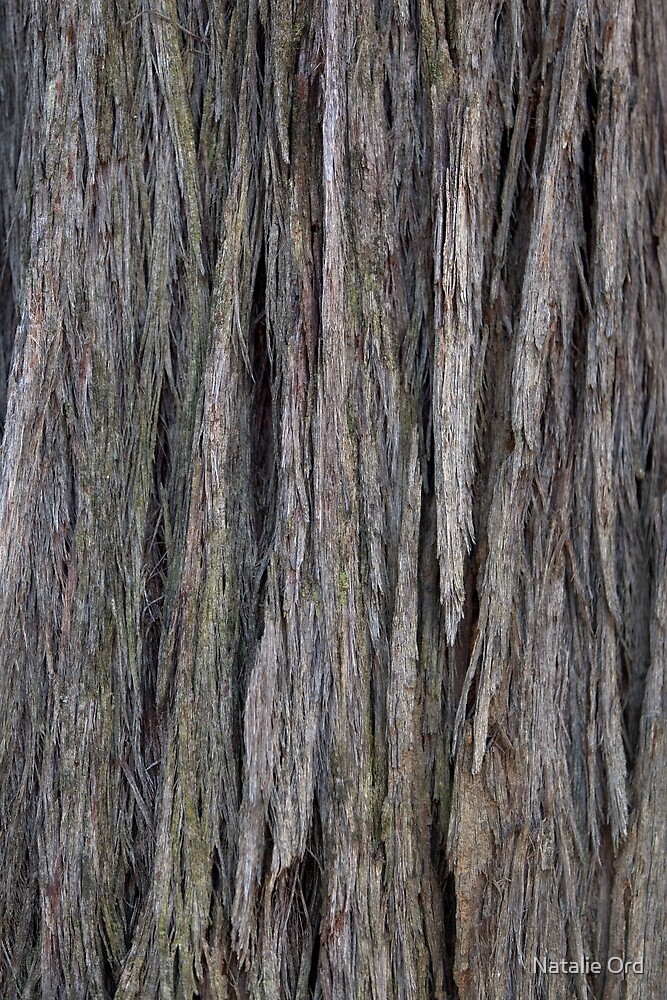The image is a high-quality, close-up of craggy, splintery tree bark, captured with remarkable detail. The vertically aligned, feathery-looking bark is predominantly a gray-brown color with streaks of green interspersed throughout. There are deep grooves in the bark, making it appear almost as if the texture is coming off the tree in thick clusters. As you move from the top to the bottom of the image, the coloration transitions from darker shades of gray with more green on top to much lighter, almost white-gray hues at the bottom, where the bark appears more separated. The entire photograph is rectangular and features the small, white text "Natalie Ord" in the bottom right corner, presumably indicating the artist's name.